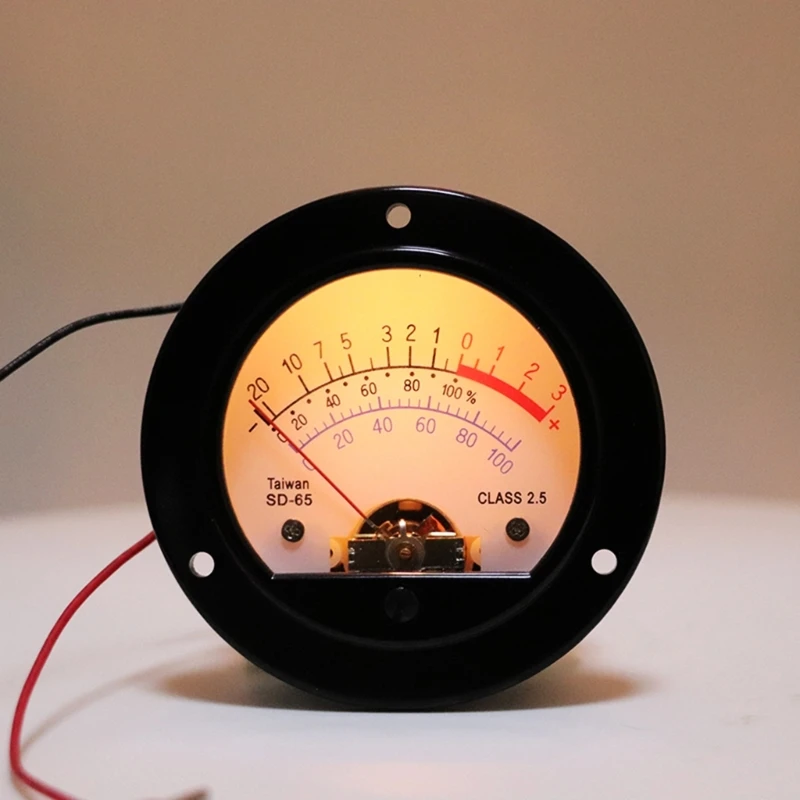This image features an electric meter with a round, black casing and a white face, positioned upright on a white surface with a matching white background. The meter, labeled "Taiwan SD-65" on the left and "Class 2.5" on the right, displays a red pointer currently set at zero. The dial includes a detailed scale: the outer arc starts at -20 on the far left, moving through 0 at the center, and extending to +3 on the far right. The values from 0 to 3 are marked in red, while the rest are in black. Below this scale, there is another set of numbers in blue, ranging from 0 to 100%. The meter is unconnected, with black and red wires extending from its back and trailing off to the left side, out of frame. The dial face is illuminated with a yellowish light, highlighting the intricate details and scale markings. This comprehensive setup underscores the meter's precision and design specificity, blending multiple color-coded arcs and numerical indicators for versatile readings.